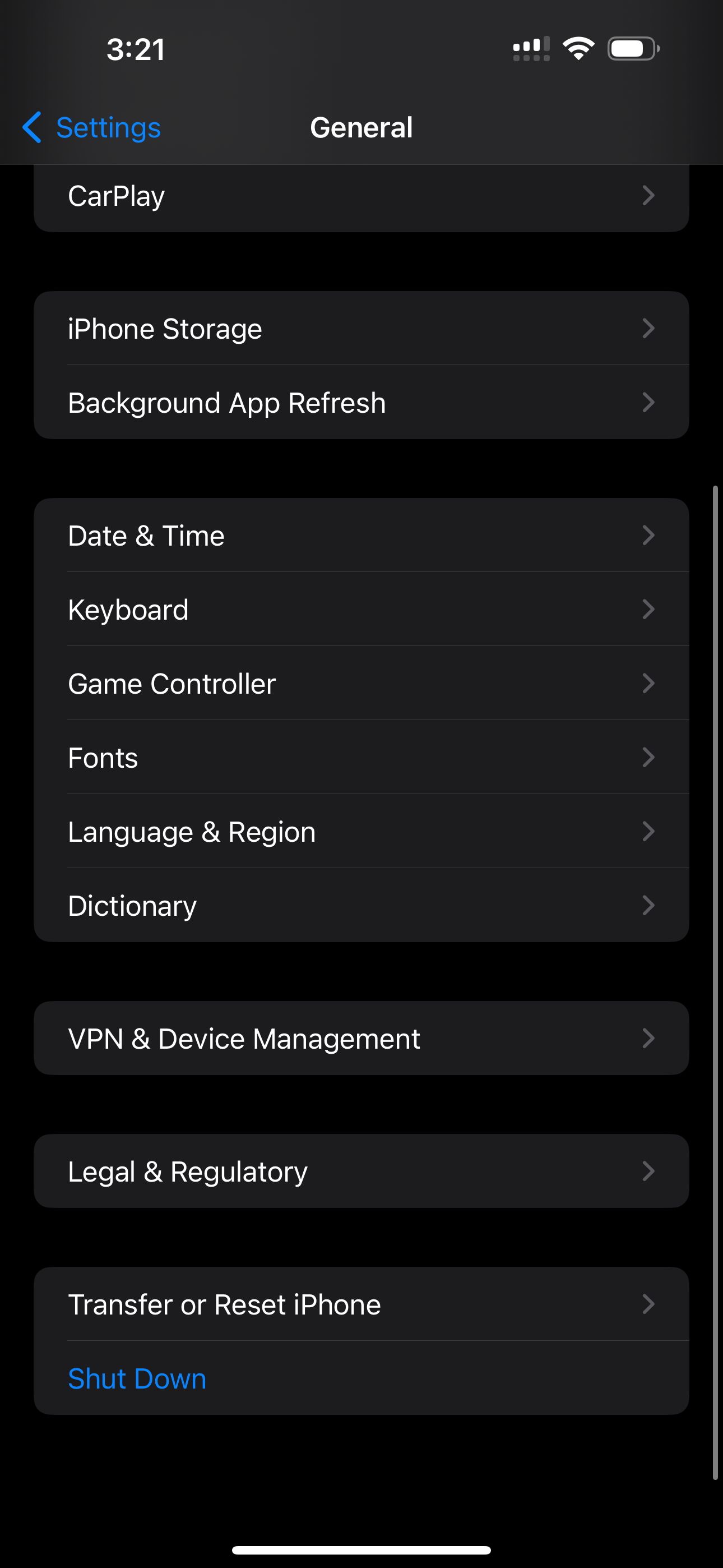This screenshot, taken from an Apple iPhone, displays the General Settings menu at 3:21 PM. The screen is scrolled to the bottom, highlighting several options:

- **CarPlay**: Integrates the iPhone with a car's infotainment system.
- **iPhone Storage**: Displays a detailed breakdown of apps, documents, pictures, and other data consuming storage space, allowing users to manage and free up space by removing unnecessary items.
- **Background App Refresh**: Manages which apps can refresh their content in the background.
- **Date & Time**: Provides options to manually set or automatically update the device's date and time.
- **Keyboard**: Customizes the keyboard layout, including positioning for left or right-handed use and text settings.
- **Game Controller**: Allows configuration of settings for connected game controllers.
- **Fonts**: Enables changes to the font style and size used throughout the device.
- **Language & Region**: Adjusts the device's language and region settings, influencing formats and input methods.
- **Dictionary**: Allows the addition of personalized words to improve typing accuracy and predictive text.
- **VPN & Device Management**: Configures VPNs to encrypt data and manage device connections securely.
- **Legal & Regulatory**: Provides important legal and regulatory information.
- **Transfer or Reset iPhone**: Options for transferring data to a new device or resetting the current one.
- **Shutdown**: A distinct blue-labeled option to completely power off the device.

This comprehensive menu empowers users to customize their iPhone settings according to their needs and preferences.